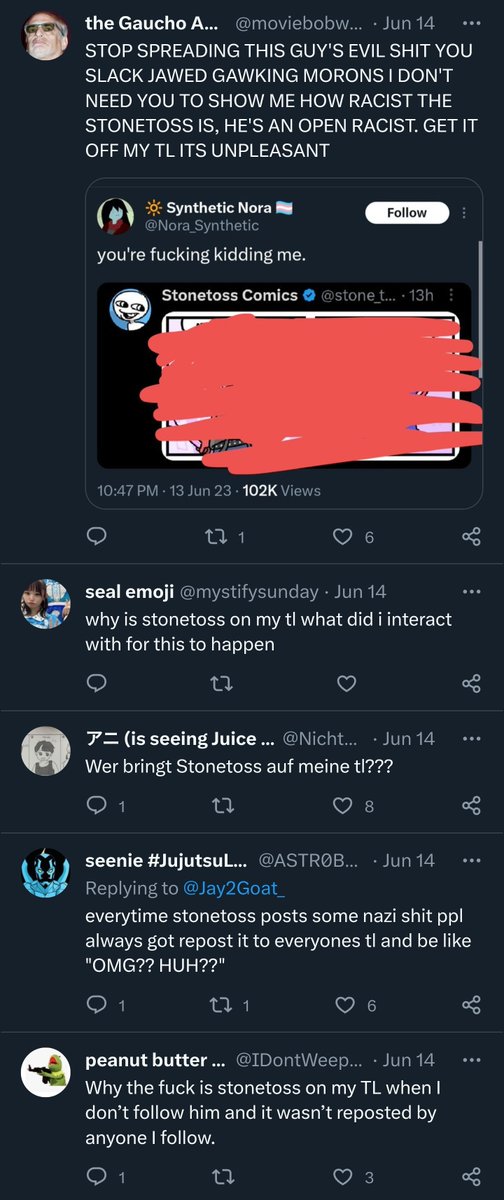This image is a vertical screenshot from a phone, displaying a Twitter thread on a dark gray background with white text. The thread consists of five posts, all discussing the comic author known as Stone Toss. Each post expresses anger towards Stone Toss, accusing his comics of being offensive.

At the top of the thread, user @TheGalchoA vehemently posts in all capital letters: "STOP SPREADING THIS GUY'S EVIL SHIT, YOU SLACK-JAWED GAWKING MORONS. I DON'T NEED YOU TO SHOW ME HOW RACIST THE STONE TOSS IS, HE'S AN OPEN RACIST. GET IT OFF MY TL, IT'S UNPLEASANT."

The subsequent four posts echo this sentiment, with users expressing confusion and frustration over why Stone Toss's content appears on their Twitter timelines. Comments like "Why is Stone Toss on my TL?" and "What did I interact with for this to happen?" highlight their collective displeasure.

Each post features typical Twitter interaction metrics, including the number of likes, retweets, and comments, indicating the engagement these posts have garnered. The screenshot captures a moment of collective outrage towards Stone Toss on the Twitter platform.